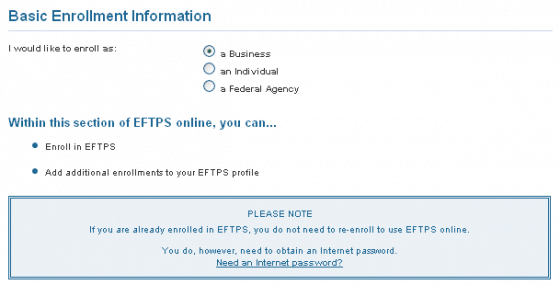Caption: 

The image provides detailed instructions for enrolling in the Electronic Federal Tax Payment System (EFTPS). The main heading, "Enrollment Information," is prominently displayed at the top. Users are given the option to enroll as a business, an individual, or a federal agency, with the example shown being a business. The section outlines how to enroll in EFTPS and add additional enrollments to an existing EFTPS profile.

A blue box with blue text highlights an important note: "Please know if you are already enrolled in EFTPS, you do not need to re-enroll to use EFTPS online. You do, however, need to obtain an internet password." Below this note, in bold text, is the question "Need an internet password?" This reiterates the reminder that if a user is already enrolled in EFTPS, re-enrollment is unnecessary for online use, but an internet password is required.